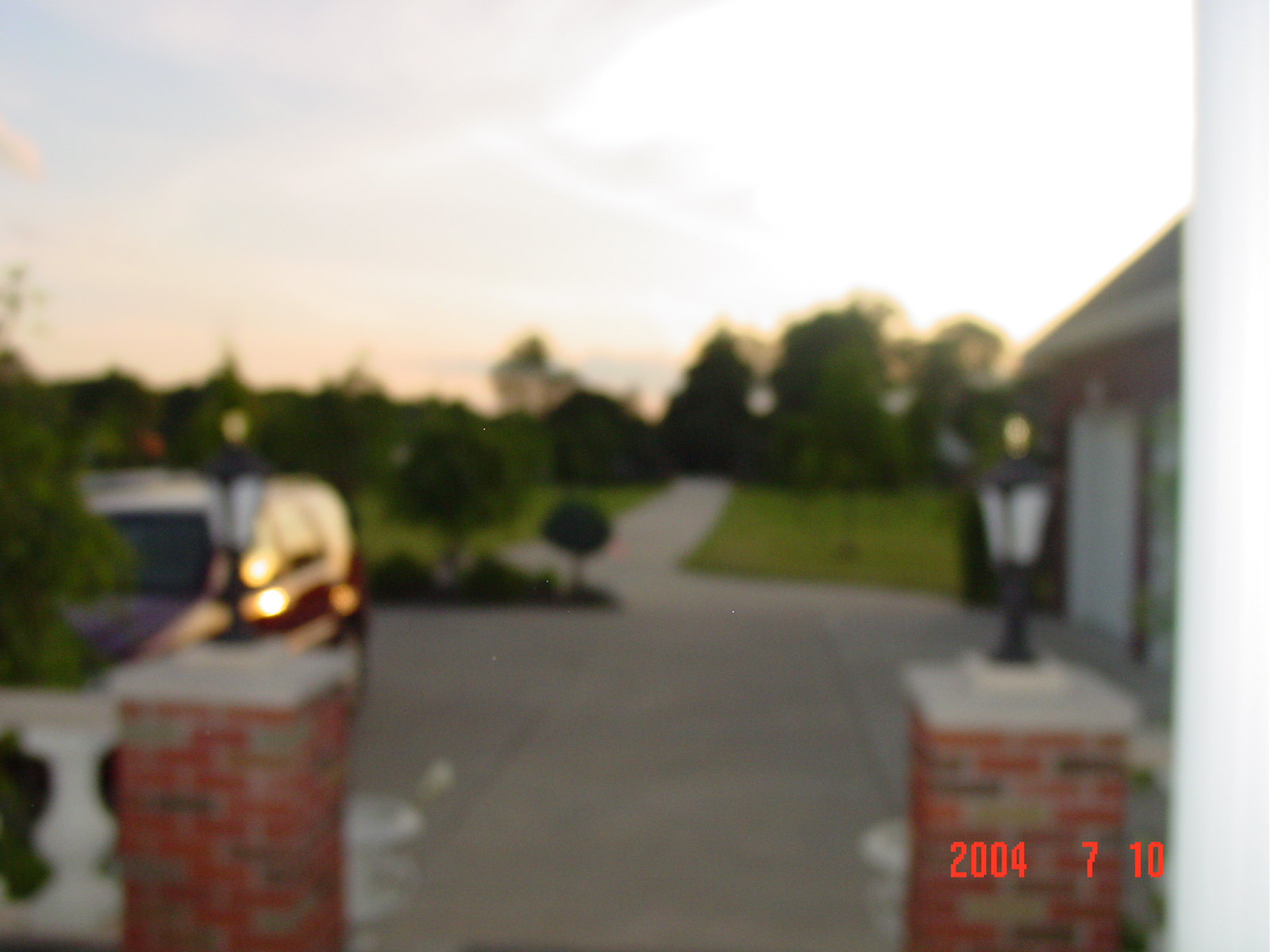In this slightly obscure and blurry photograph taken with a digital camera, we see the front yard of a house, timestamped July 10th, 2004, in the bottom right-hand corner. The image is framed by two short red brick pillars with unlit black lanterns on top. A large, flat, circular driveway, gray in color, dominates the foreground, extending into the distance. To the left, there's a parked, dark red vehicle, possibly a van or station wagon, reflecting the sun. Behind the car, some topiaries or garden plants are visible. On the right side, part of the house comes into view, featuring at least one or two white garage doors indicative of a double-sided garage that can accommodate several vehicles. The brown-roofed house is surrounded by lush green lawns and numerous trees, with a long walkway or road extending into the neighborhood. The scene appears to be captured around sunset, with a serene suburban ambiance.